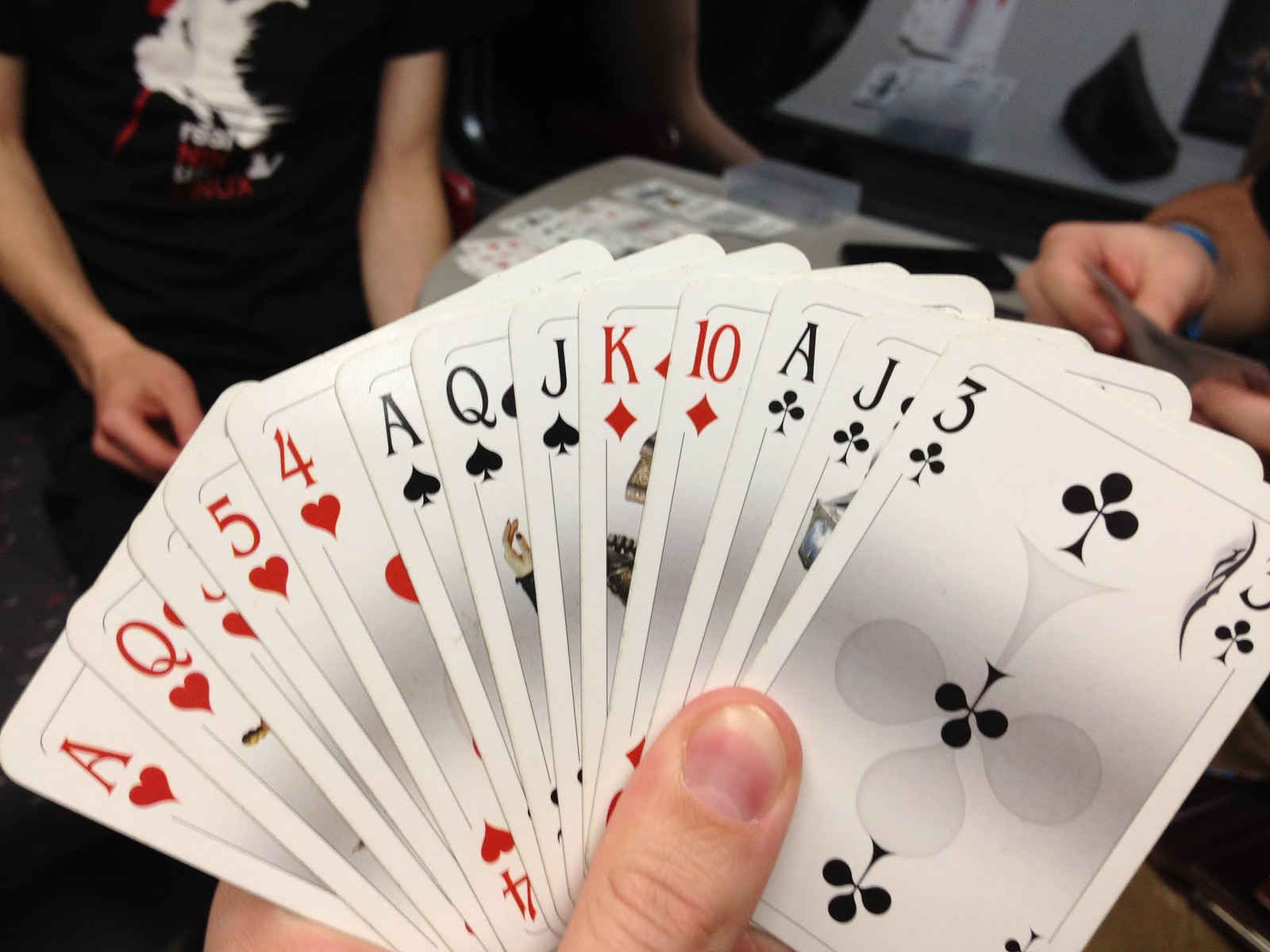In the image, a card game is in full swing. At the bottom center, a well-groomed left thumb, with its short, clean-cut, non-polished nail, possibly belonging to a Caucasian individual, is visible. The thumb is part of a hand holding a spread of playing cards, which from left to right, includes an Ace of Hearts, Queen of Hearts, Jack of Hearts, Five of Hearts, Four of Hearts, Ace of Spades, Queen of Spades, Jack of Spades, King of Diamonds, Ten of Diamonds, Ace of Clubs, Jack of Clubs, and Three of Clubs. 

Adjacent to the hand, in the bottom right corner, small brown and dark objects are partially discernible. The cards held are plain white with a narrow black border. 

In the top right corner, a pair of hands emerges from an orangeish-brown sweater with a hint of blue, possibly a cuff, suggesting the presence of another player. Behind these hands, a dark area is followed by a white wall, featuring a table with dark objects and what appears to be the back of some boxes, all on a gray surface.

At the center, the hands rest on a table, amid other laid-out cards. A mirror in the background reflects another player in the upper left corner, who is wearing a black t-shirt with a white and red figurine design. Additional cards and a smartphone are also visible on the table near the player in the top right. The mirror provides a broader view, capturing the third player's arm and the general game setup, enhancing the image's complexity and depth.